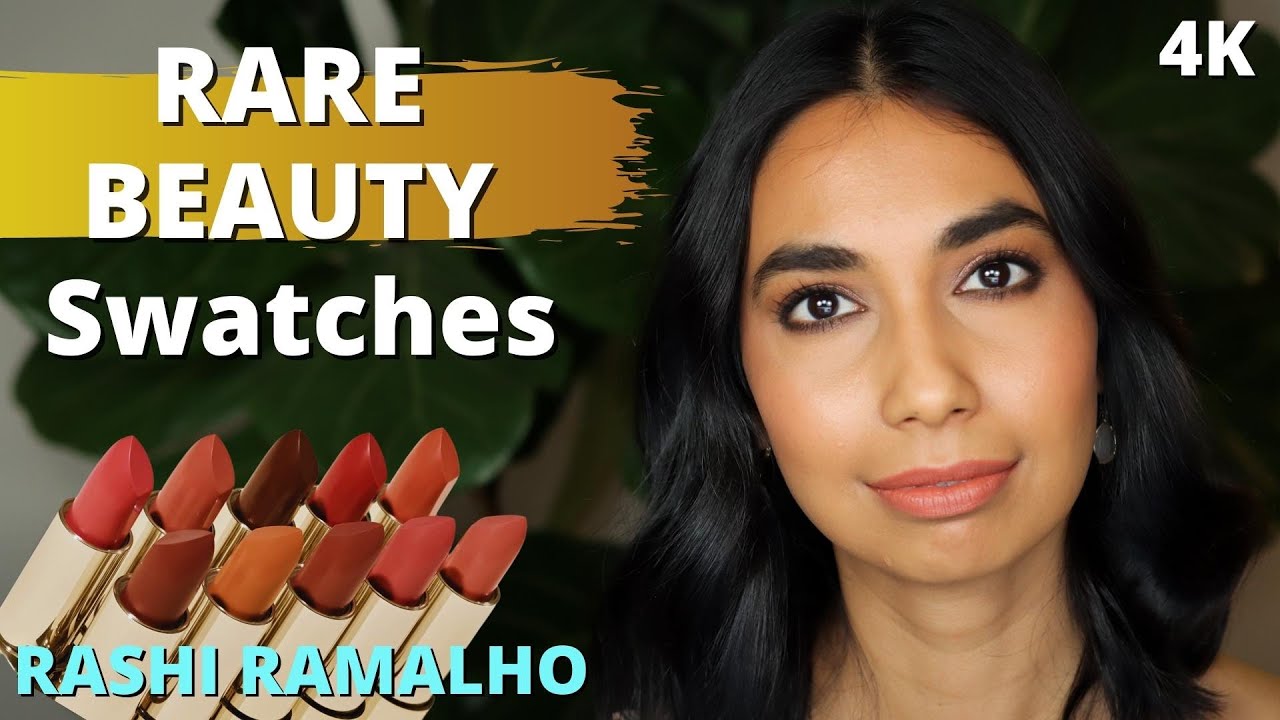The image appears to be an advertisement or a video thumbnail for a makeup line by Rashi Ramalho. The top left corner features the text "Rare Beauty Swatches" in white, with a streak of yellow behind it and a background accent of green. Below this text are ten lip glosses in various colors, displayed in a row. Over the lip glosses, the name "Rashi Ramalho" is printed in blue letters. The woman on the right side of the image appears to be a South Asian or Indian model with a brown complexion, long black hair, dark brown eyes, and dark eyebrows. She is wearing a light red lipstick and is looking directly at the viewer. Notably, the upper right corner of the image displays "4K," suggesting high-definition quality. The overall setup includes professional lighting, and the background appears to be softly blurred with possibly a plant visible.